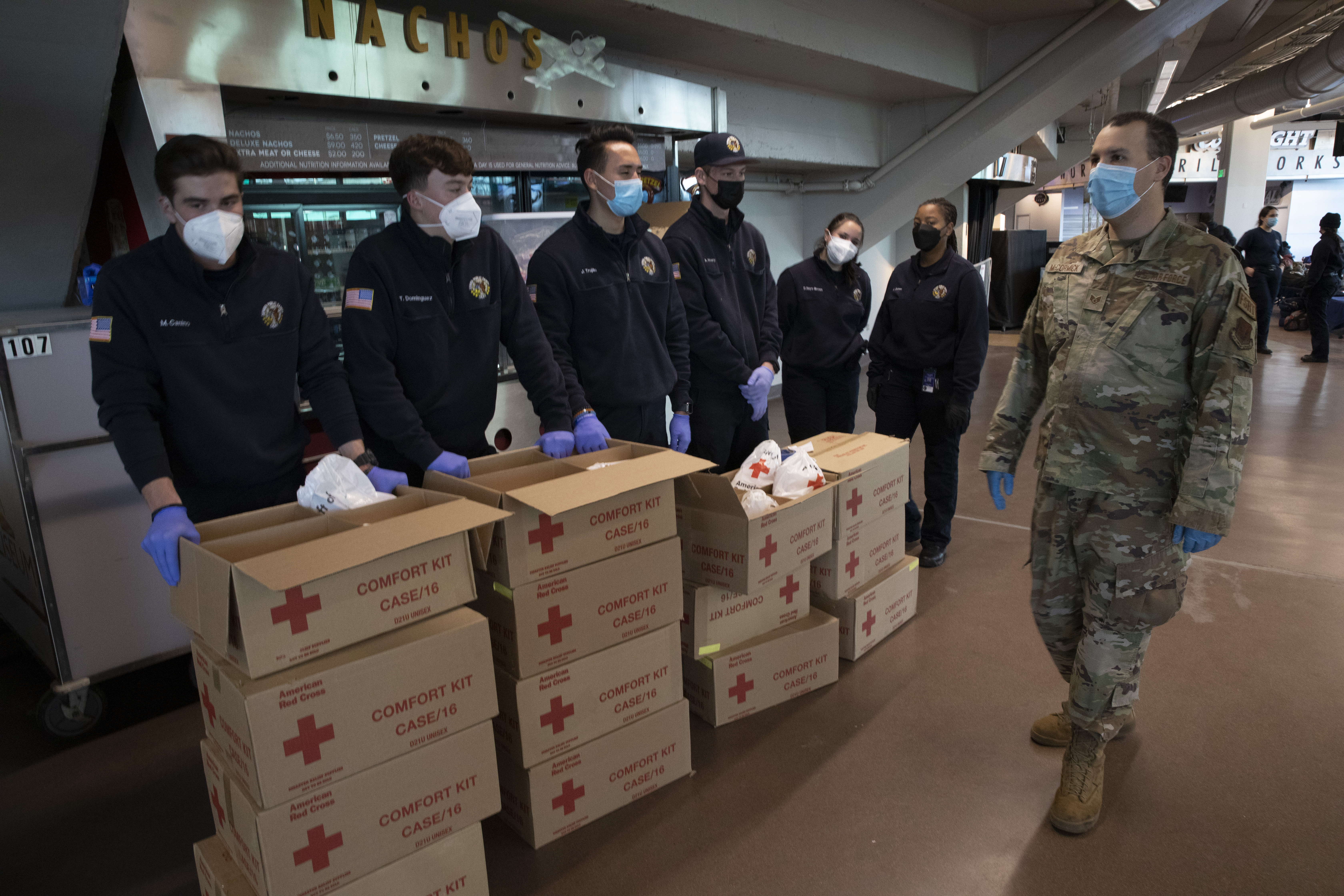This photograph depicts a group of individuals, both men and women, in an indoor setting that resembles a stadium or possibly an airport terminal, identifiable by the concession sign in the background offering "nachos" for $6.50. In the foreground, a soldier in a desert camouflage uniform, complete with brown combat boots, a mask, and blue gloves, is inspecting Red Cross comfort kits. Surrounding him are several people in black quarter zips, each embroidered with their names and an American flag on the sleeve. These individuals, also donned in masks and medical-like purple gloves, appear to be distributing the comfort kits, which are neatly stacked in cardboard boxes labeled "case 16." The scene suggests a coordinated effort likely related to a relief or support mission, underscoring the meticulous safety measures in place during the COVID-19 pandemic.